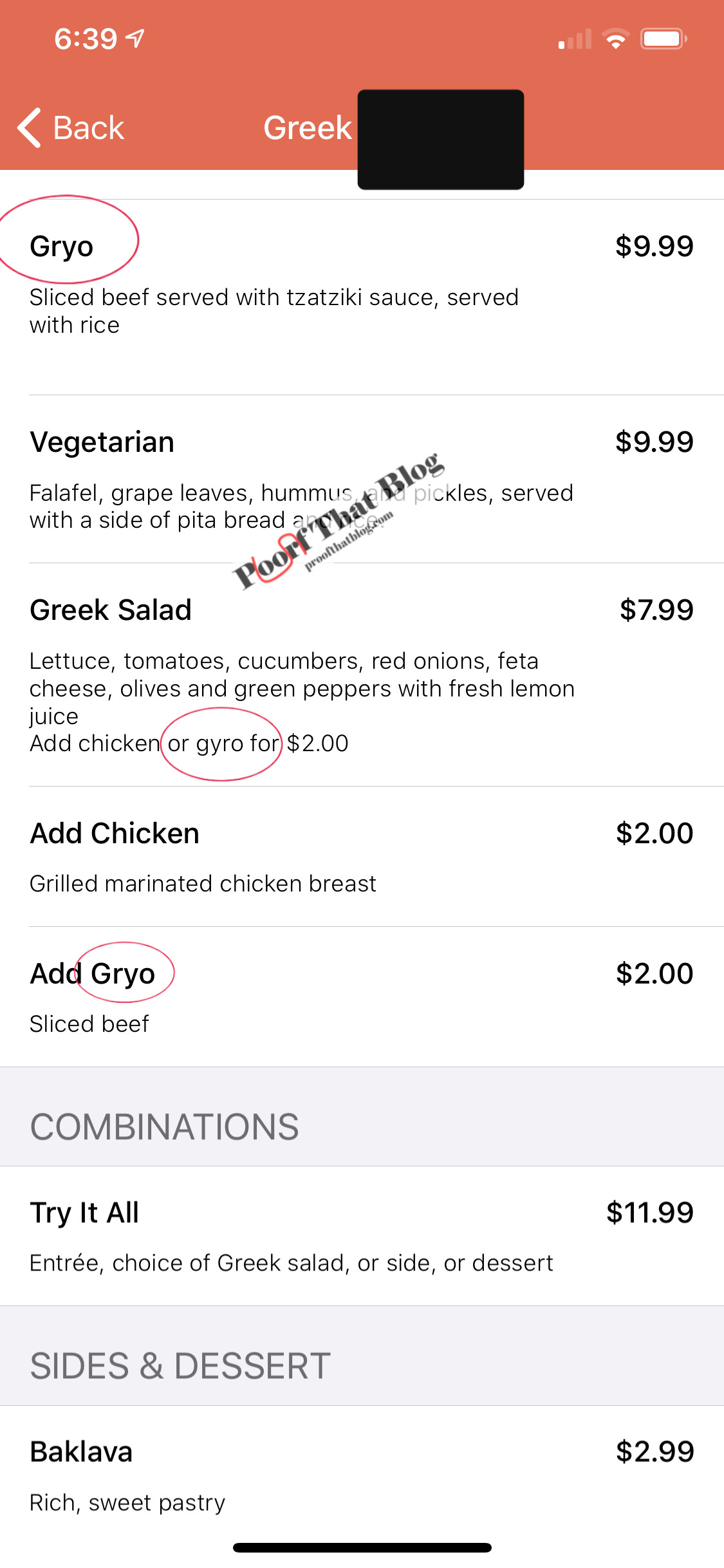The image captures a smartphone screen where someone is in the process of ordering Greek food from an online menu. At the top of the screen, the status bar displays an orangish-red backdrop with the current time noted as 6:39, alongside a white paper airplane icon. The battery indicator appears to be fully charged, represented by a solid white battery icon, and various other common notification icons are visible.

Just below the status bar, there's a back button pointing to the left, facilitating navigation. The word "Greek" headlines the menu, though a black rectangle obscures some adjacent text, likely for privacy reasons pertaining to the restaurant's name.

Directly beneath this title, a highlighted menu item, "Gyro," is encircled in red. The description reads: "Sliced beef served with tzatziki sauce, served with rice," priced at $9.99. The menu proceeds to list "Vegetarian" options, specifying dishes such as falafel, grape leaves, hummus, and pickles, each served with a side of pita bread.

An off-centered stamp stating "proofthatblog.com" is conspicuously marked across the menu, albeit misspelled as "P-O-O-R-F" instead of "P-R-O-O-F." Additional menu items are circled further down the page, indicating the user's selections or points of interest.